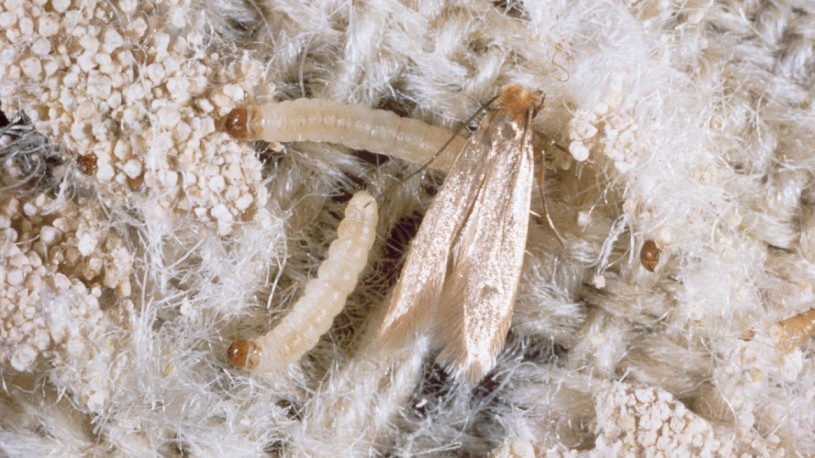The horizontal rectangular photograph depicts an enigmatic assortment of objects in various shades of brown and white. Dominating the left side are clusters of small, round, oatmeal-like particles arranged into rectangular shapes. On the right side, the bottom section features similar clusters, while the upper right is occupied by a white, fuzzy area resembling a mass of fibers, behind which thicker, square fibers are visible. Centrally positioned are four elongated, tapering shapes, possibly caterpillars, lying amid this scene with a dark brown background behind them. The overall impression is ambiguous, suggesting a mix of organic and possibly fabric materials, perhaps viewed at a microscopic level.